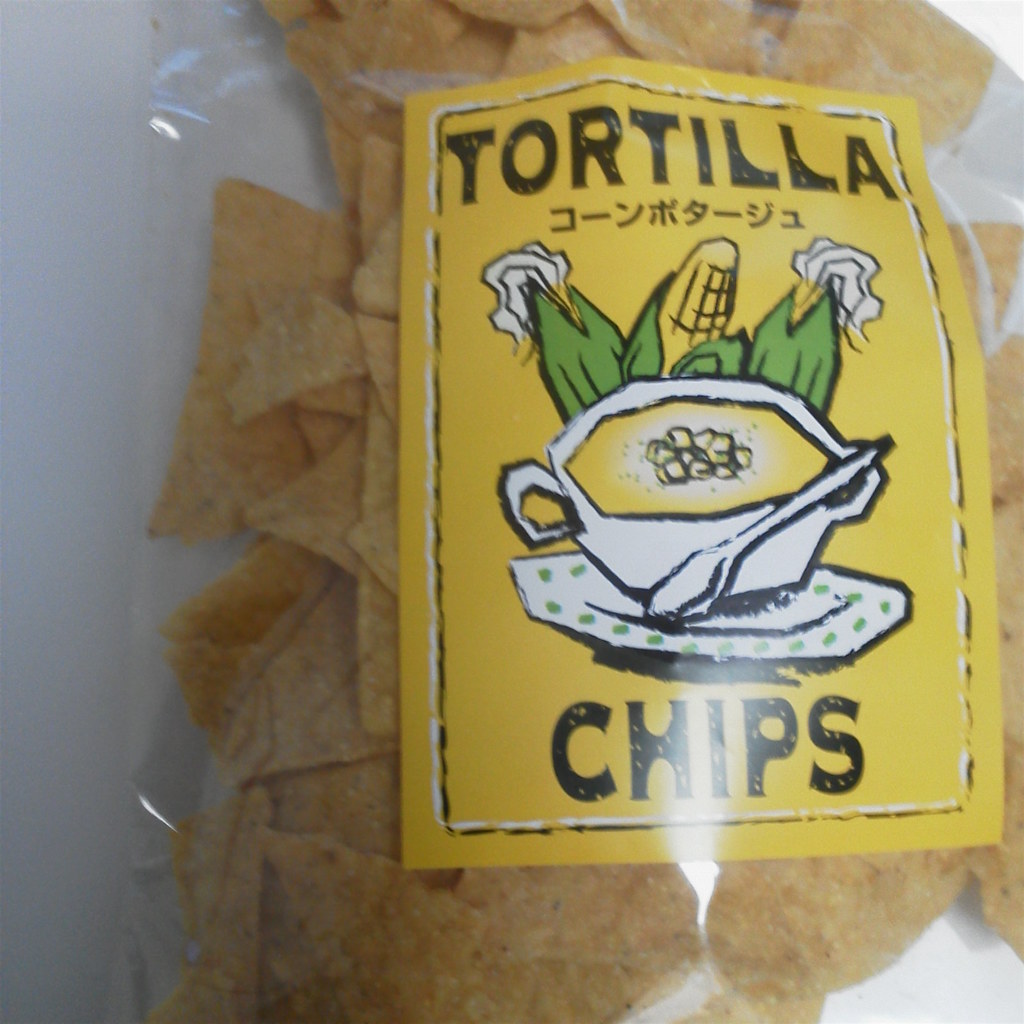The image captures a packet of brown tortilla chips encased in a transparent plastic bag. The bag features a large yellow rectangular label at the center. The top of the label boldly displays the word "Tortilla" in black lettering, while the bottom reads "Chips," also in black text. In between, there is a detailed image showing a white bowl atop a white plate with a white spoon. The bowl appears to contain a golden liquid, possibly guacamole. Prominently rising from the bowl is an ear of corn, surrounded by green stalks, with the corn itself depicted in yellow. The entire design is framed by a border that alternates between black and white. The dominant colors on the packaging, aside from the transparent material and the brown chips, include yellow, green, black, and white.